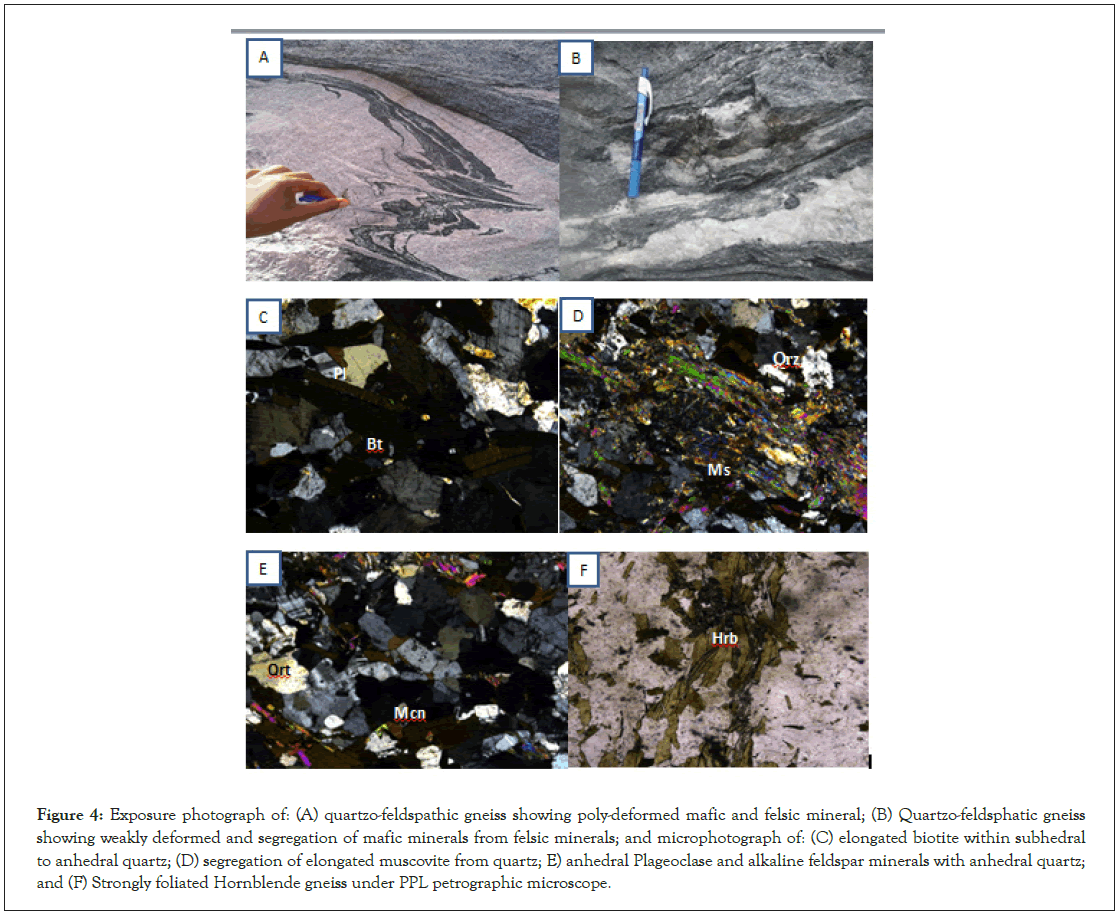This detailed image, reminiscent of those found in science textbooks, showcases six labeled photographs (A through F) depicting various rock formations and mineral deposits, likely related to exposure therapy of quartz phenographic genesis. Each photograph is primarily composed of gray, black, and tan tones with sparse accents of green, red, and blue. The first image (A) features a hand pointing at different slates, emphasizing quartzofeldspathic gneiss. The second image (B) includes a pen for scale, also highlighting quartzofeldspathic gneiss. The third image (C) displays elongated biotite stones in various shades of gray and beige. The fourth image (D) shows broken granite with labels indicating the segregation of elongated muscovite from quartz. The fifth image (E) presents further fragmentation of the slates or mineral deposits, identified as anhedral plagioclase and alkaline feldspar. The final image (F) zooms in on the minerals, illustrating strongly foliated hornblende gneiss. An explanatory figure at the bottom provides detailed descriptions for each photograph.